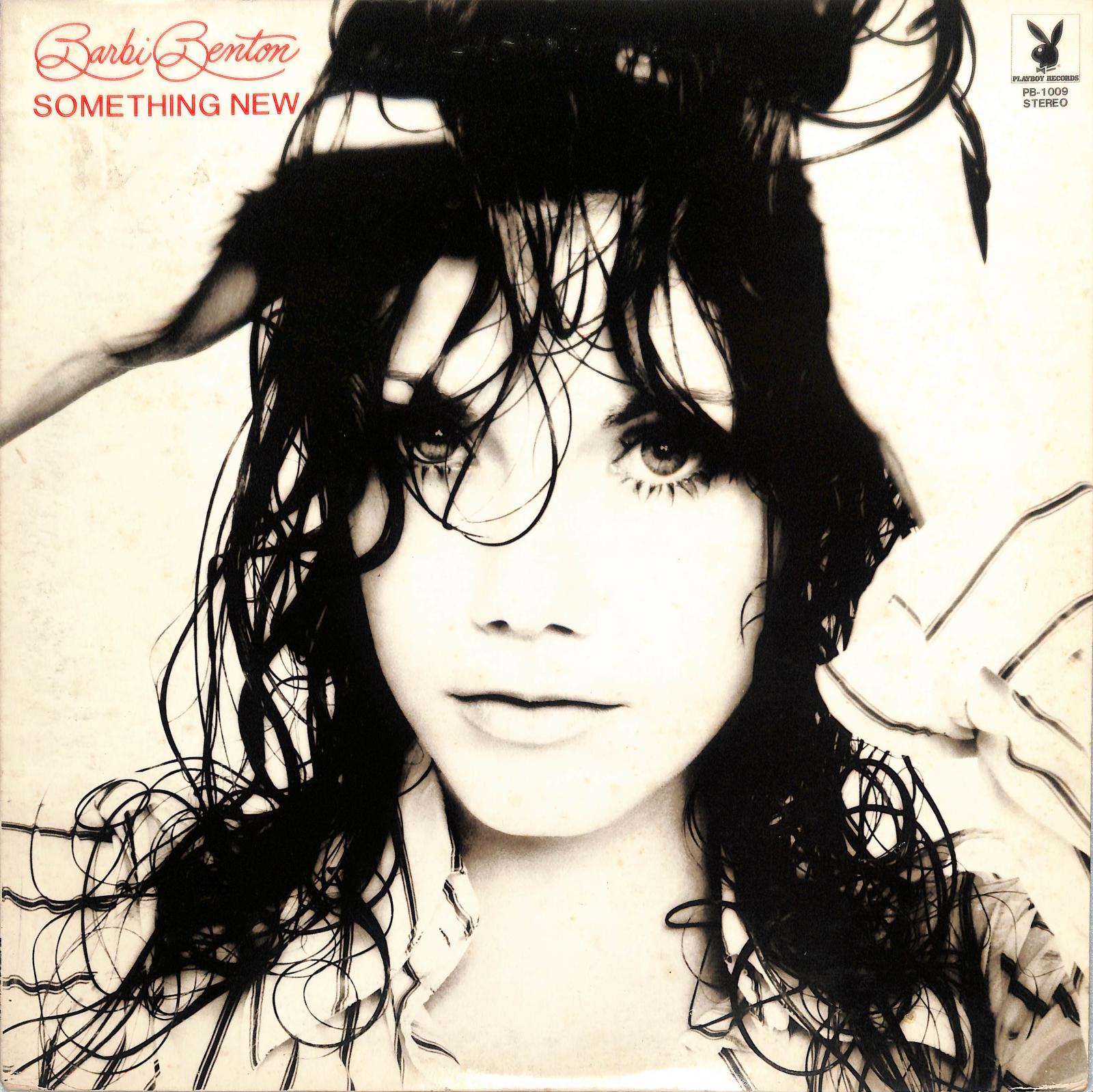The image is a vintage vinyl record cover with an aged appearance, characterized by a whitish center and yellowing edges. The top left corner features the name "Barbi Benton" in red cursive script, with the phrase "Something New" in capitalized red font below it. In the upper right corner, there is a black Playboy bunny logo within a square outline, under which it says "Playboy Records" and in smaller text "PB 1009 Stereo."

The cover displays a young woman from the neck up, with parts of her shoulders visible. She has long, wet black hair that she is running her hands through, positioned atop her head. Some strands of her hair fall over her forehead. The woman has long eyelashes, pale skin, and a wide nose. Her expression is direct, as she stares at the viewer with slightly parted lips. She is wearing a white and black striped shirt that is open, with the image cutting off just above her chest. The photo is in black and white, contributing to the vintage aesthetic of the cover. There is no discernible background, keeping the focus entirely on her face and upper body.